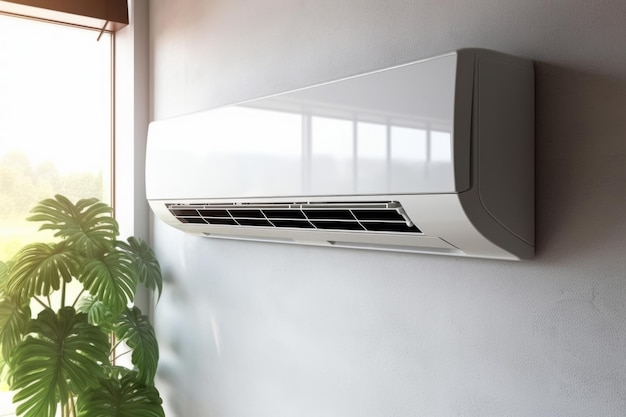The image showcases a sleek, wall-mounted air conditioner with a minimalist, rectangular design. The unit, entirely white, has a flat front with ventilation slats located at the bottom. Its underside has a slight rounded curvature, adding to its modern aesthetic. The air conditioner is mounted on a pristine white wall. In the upper left corner of the image, part of a window with a wooden top frame is visible, along with the upper portion of a leafy green plant, perhaps a tree, encroaching from the bottom left. The close-up nature of the photo brings out the details and clean lines of the air conditioner, making it the focal point of the composition.